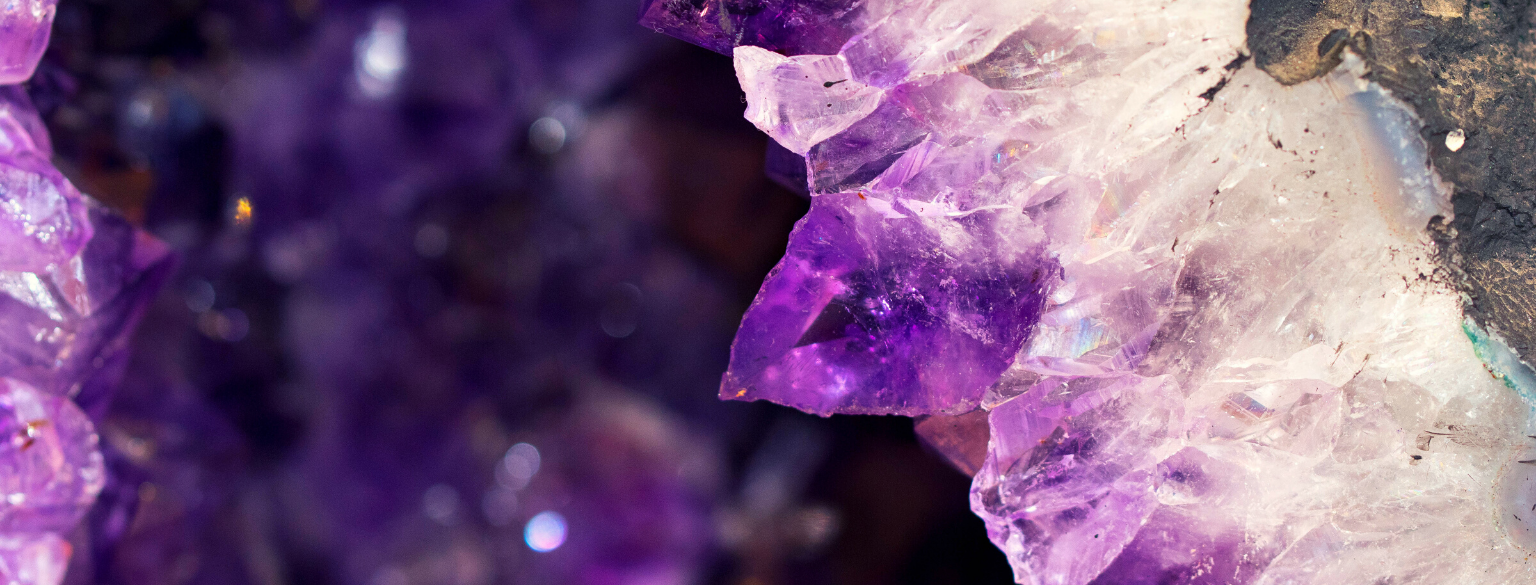In this photo, a stunning array of crystals and minerals is showcased, seemingly situated in a cave. Dominated by purple amethyst and white quartz, the crystals are illuminated by sunlight, which causes them to sparkle and appear vibrant. The background of the image is a blurred, dark expanse, providing a stark contrast to the sharp, glittering crystals in the foreground. The amethyst formations on the left are prominent and jagged, while on the right side, some white crystal, possibly quartz, adds to the striking display. The entire scene gives the impression of a close-up view of a geode's interior, with its beautiful and sharply defined crystalline structures catching the light and creating a mesmerizing visual effect.